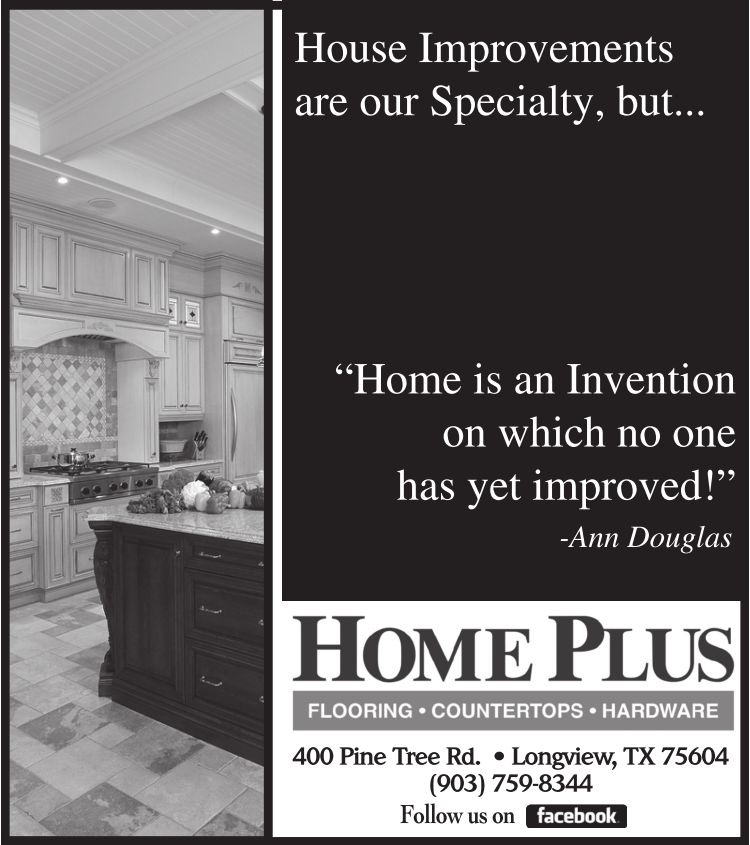This black and white advertisement for HomePlus features a highly detailed depiction of a kitchen on the left and informative text on the right. On the left side, there is a black and white photo showcasing a modern kitchen with a tile floor, a central wooden island equipped with drawers, and a marble tabletop. The background reveals neatly arranged cabinets, emphasizing the kitchen's elegant design.

On the right side, the ad displays a quote in white text against a black background: "Home is an invention on which no one has yet improved" - Ann Douglas. Below this quote, the HomePlus logo is prominently featured alongside their specialties listed in a gray background with white text: Flooring, Countertops, and Hardware. The ad also provides the company's address, 400 Pine Tree Road, Longview, Texas 75604, and contact number, 903-759-8344, urging viewers to follow them on Facebook. This comprehensive ad effectively merges visual appeal with detailed information, highlighting HomePlus' dedication to home improvement.